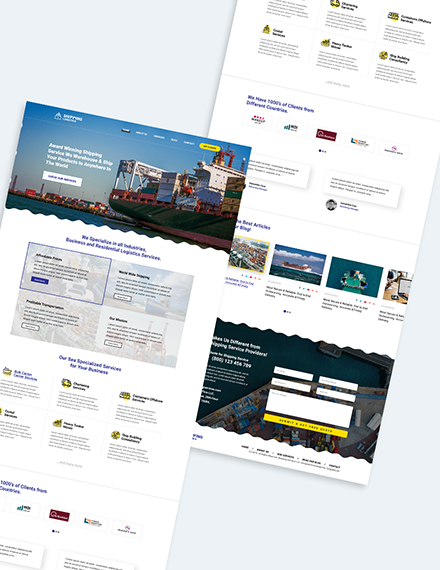The screenshot features two slanted website pages, tilted to the right. The most prominent page is positioned in the bottom left corner and appears to be a cargo shipping website. At the top of this page, a picture showcases a cargo ship loaded with containers in its hull, along with several other cargo ships docked in a harbor. To the right of the ship image, there's a striking yellow button, and to the left, a white button.

The lower border of the ship image has a wavy design. Below it, there is a four-panel chart with blue titles, though the text is difficult to read even when zoomed in. This section of the webpage has a white background and several sections adorned with icons.

The second page, slightly visible behind the first, also features a white background. It seems to be a continuation of the first page. This page displays a row of logos and features articles related to cargo ships towards the bottom. Some articles include heart ratings. At the very bottom of this webpage, there's a footer section with a form that requires a name and message, along with a yellow "Submit" button.